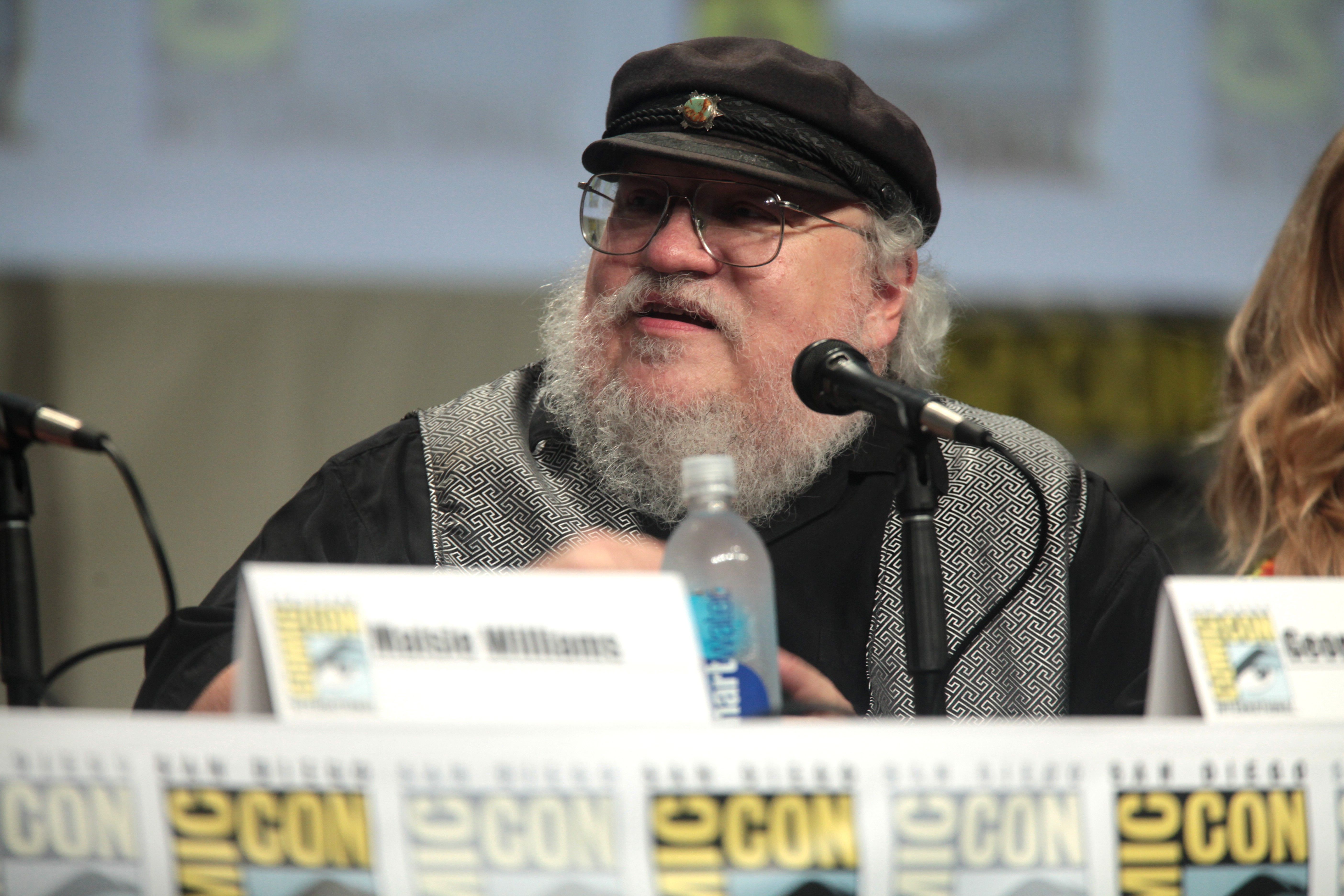The image is of George R.R. Martin at a Comic-Con event, presumably discussing Game of Thrones. He is seated at a conference desk with a Comic-Con banner in front that partially spells out "MIC... CON." Martin, a large man with a gray beard and mustache, is wearing his signature black flat cap, glasses, a black shirt, and a black and white vest. In front of him on the desk are a bottle of Smart Water, a microphone, and a piece of paper likely displaying his name. Next to him sits Maisie Williams, identifiable by her long blonde hair and visible arm.